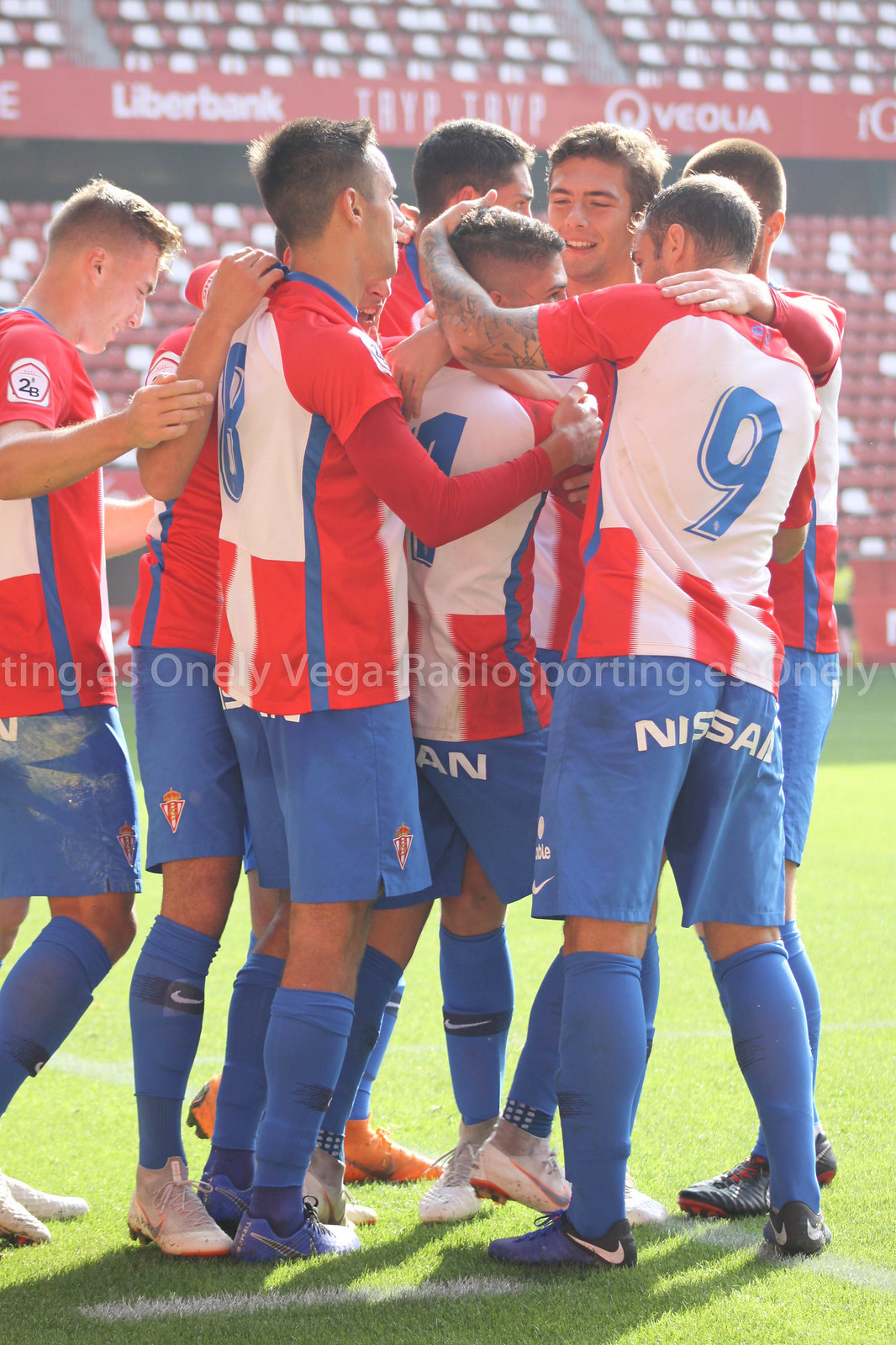This detailed photograph captures the celebratory moment of a soccer team, presumably just after scoring a goal. The players, dressed in white jerseys with red stripes towards the waist, red shoulders, and light blue numbers, are seen hugging each other in the middle of a green pitch with white chalk lines. The team's uniform also features light blue shorts and socks. The background reveals empty red and white bleachers, highlighting the isolation yet focus on the players' joyous moment. The image prominently displays light white text reading "only vega-radiosporting.es" in the midst of the scene. On closer inspection, the shorts show an advertisement for Nissan. The photograph, taken on a sunny day with sunlight streaming from the right and casting shadows to the bottom left, showcases the players in high spirits, with several identifiable numbers, such as nine and eight, facing away from the camera. One player, distinguishable by his short brown hair, faces the camera but his jersey is obscured. The overall mood is one of triumph and camaraderie on an otherwise quiet soccer field.